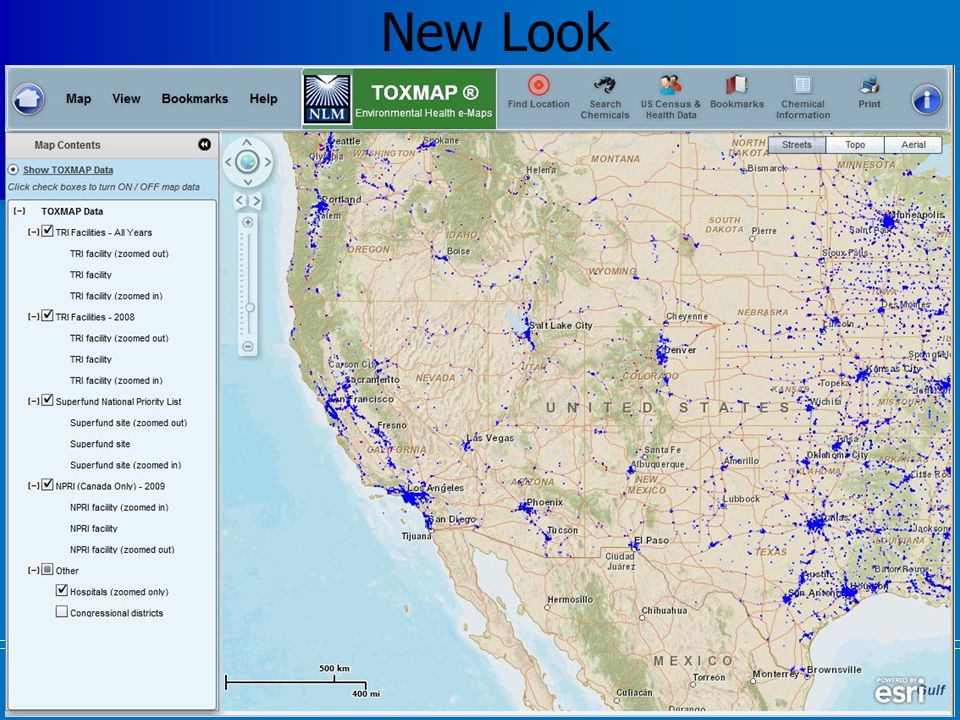The screenshot depicts the redesigned interface of an application called "TOXMAP," developed for environmental health and e-mapping purposes. The header features a gradient background transitioning from indigo to light blue, with the text "New Look" prominently displayed in black font. Beneath this header lies the main application window showcasing several elements.

In the top section of the application window, a green rectangle is slightly off-center. It contains the app's title, "TOXMAP®," alongside descriptive text stating "Environmental Health e-Maps." Adjacent to this, on the left, is the "NLM" logo, characterized by a blue background and white sunburst lines.

The menu bar is arrayed with various buttons and icons: 
- "Home" (white house symbol on a blue button)
- "Map"
- "View"
- "Bookmarks"
- "Help."

Following this, a toolbar features icons and labels for:
- "Find Location" (target icon)
- "Search Chemicals" (binoculars icon)
- "U.S. Census and Health Data" (two people icon)
- "Bookmarks" (open book icon)
- "Chemical Information" (notepad icon)
- "Print" (printer icon).

On the left sidebar, users can interact with options such as "Map Contents" and "Show TOXMAP Data." Below these options is a collapsible menu displaying hierarchical data labels like:
- "TOXMAP Data"
- "TRI Facilities All Years"
- "TRI Facilities 2008"
- "Superfund National Priority List"
- "NPRI Canada Only 2009"
- "Other."

The central panel showcases a map of the United States, primarily focusing on the Midwest to California. The map is dotted with blue points representing various data points spread across these regions, providing a visual overview of environmental health data collected by the application.